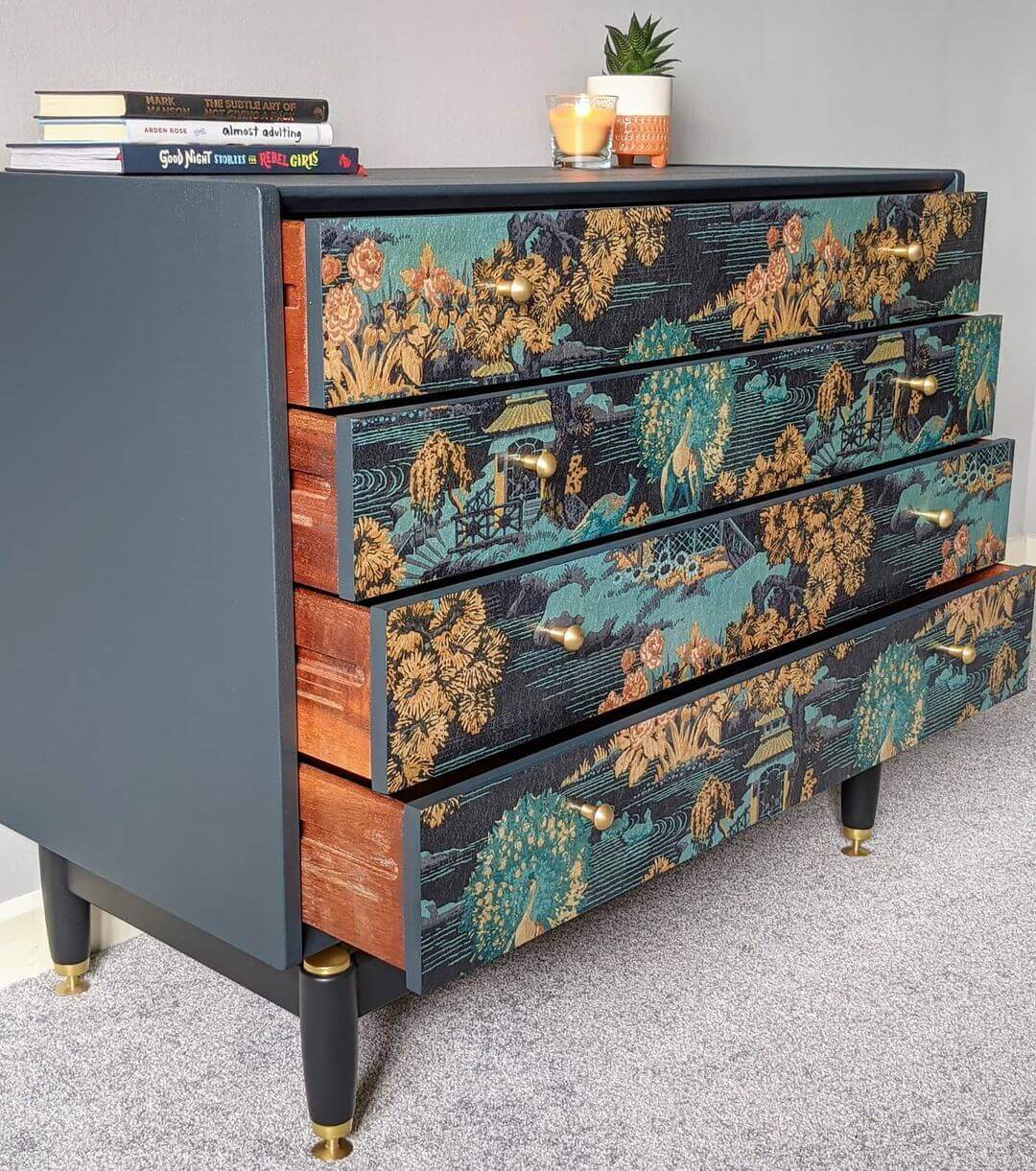The image depicts a four-drawer dresser adorned with detailed Asian art motifs, including chrysanthemums, other flowers, and pagodas. The dresser rests on a gray carpet and features four legs accented with brass ends. The drawers are painted in shades of blue, dark blue, and beige-orange and are fitted with small brass handles. The intricate teal patterns and golden handles complement the overall artistic theme.

On top of the dresser, which is painted a dark slate gray, there are three stacked books placed on the left side: a gray book at the bottom, a white book in between, and a brown book on top. The text on the books mentions "Good Night" and "Rebel Girls." To the right side at the top of the dresser, there's a small yellow candle that is lit and a plant in a holder, possibly a cactus. The dresser’s top contrasts with its white upper surface and brown underscored base. The dresser shows detailed leaf motifs set against blue and dark blue backgrounds, completing its ornate appearance.